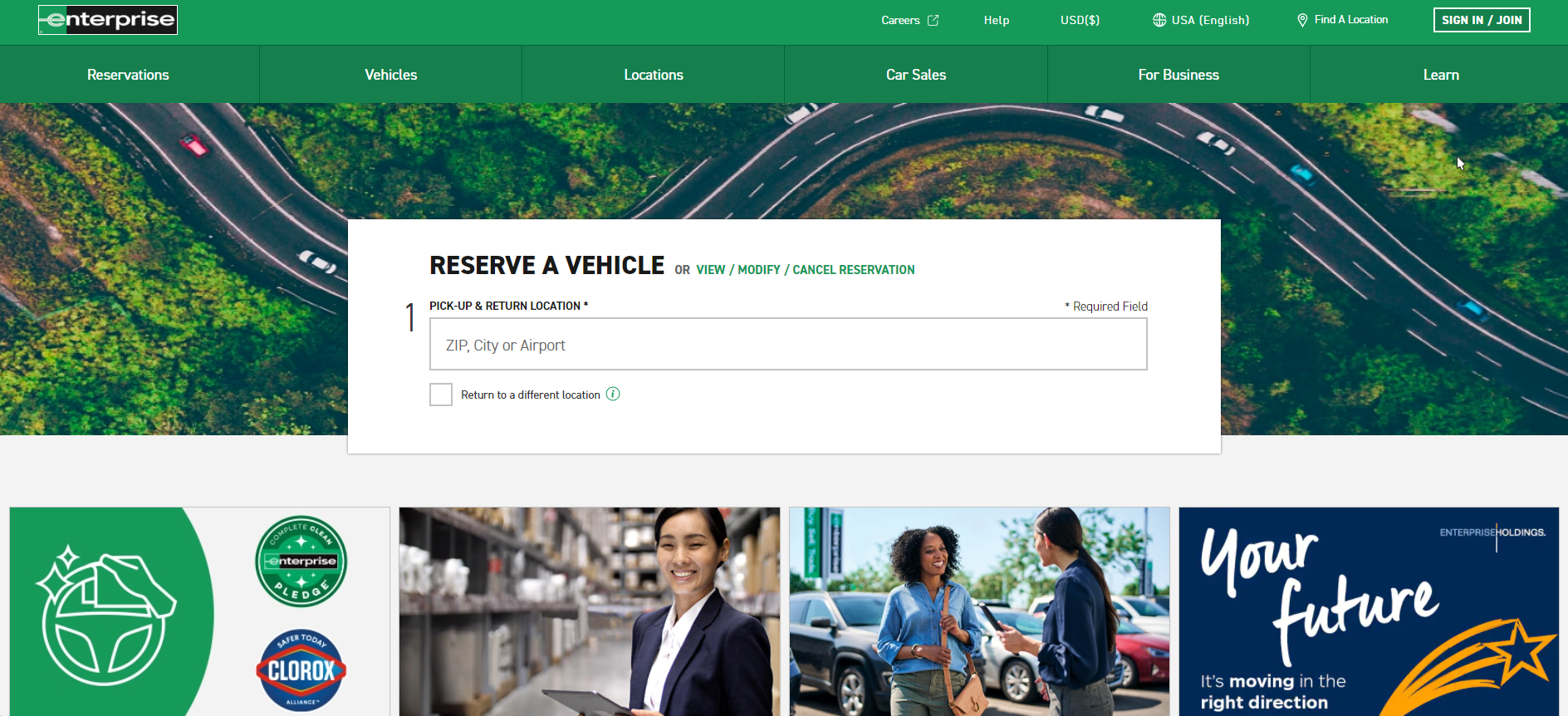This image is a detailed screenshot of the Enterprise Rent-A-Car website. In the top left corner, the company's logo, "Enterprise," is prominently displayed. Adjacent to the logo, various navigational links are available. In the far right top corner, there are sign-in and join buttons, with a 'Find Location' button positioned just to their left.

Dominating the middle section of the screenshot is a large overhead image depicting a winding road, populated with cars and surrounded by lush trees. Centrally placed within this image is a reservation section featuring a prominent search bar where users can enter their ZIP code, city, or airport to find available vehicles.

Beneath this main image, there are four smaller pictures. One image showcases sponsor logos, including Clorox. Another displays a businesswoman smiling. A third image features two women engaged in a cheerful conversation in a parking lot. The final image, located in the bottom right corner, depicts a yellow shooting star accompanied by the caption, "Your Future. It’s Moving in the Right Direction."